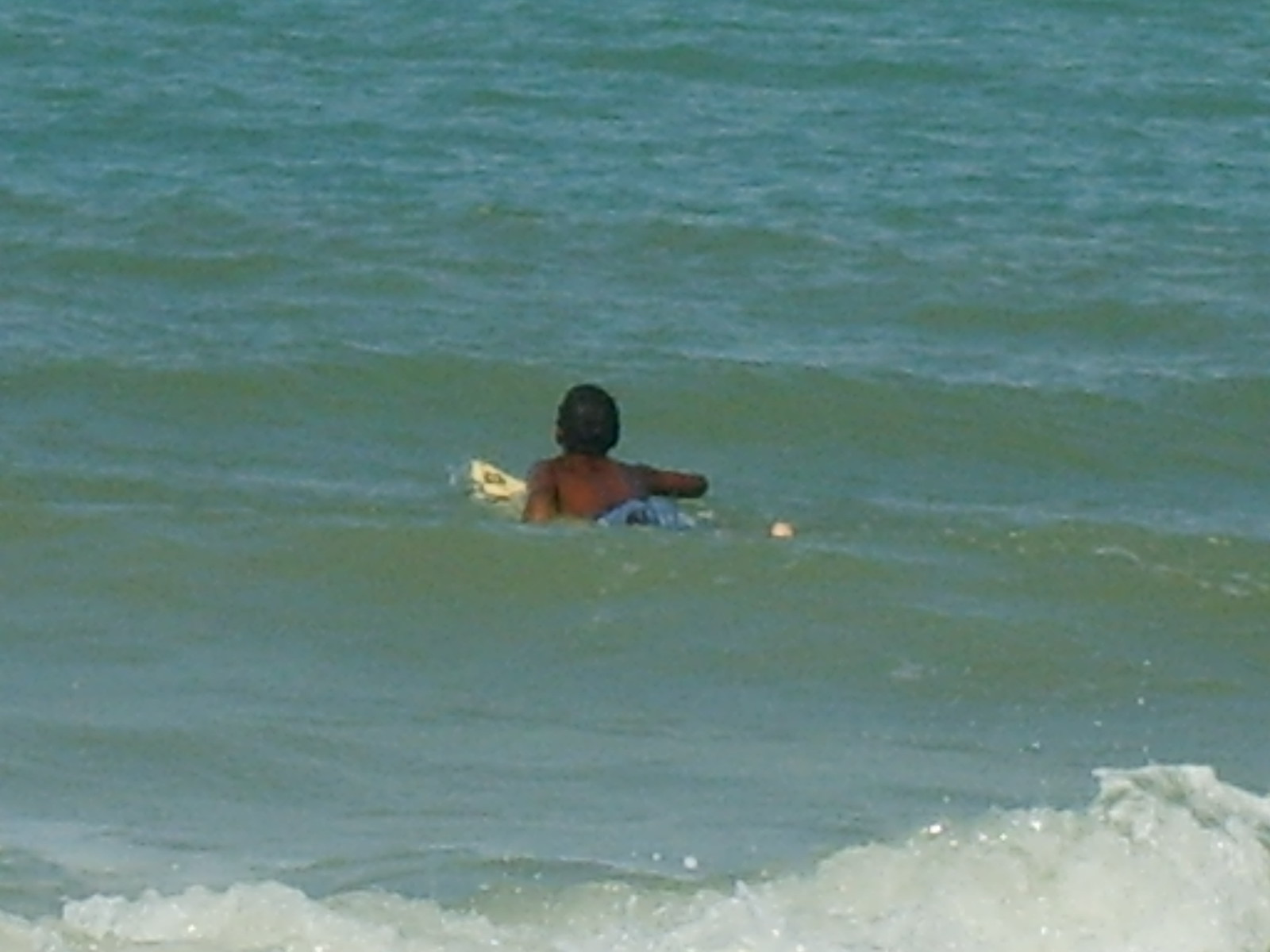In this grainy, poorly lit photograph, an African American individual is seen paddling out to sea on a tan surfboard, which is mostly submerged beneath dark blue-green, slightly choppy waters. The person's short black hair and blue swimming trunks are visible as they lay on their stomach on the surfboard, with their arms extended forward, facing away from the camera. In the background, the ocean features white, foamy waves breaking near the front of the image. The person's foot can just barely be seen sticking out of the water, highlighting the overall calmness of the sea with only modest ripples and splashes near the shore.